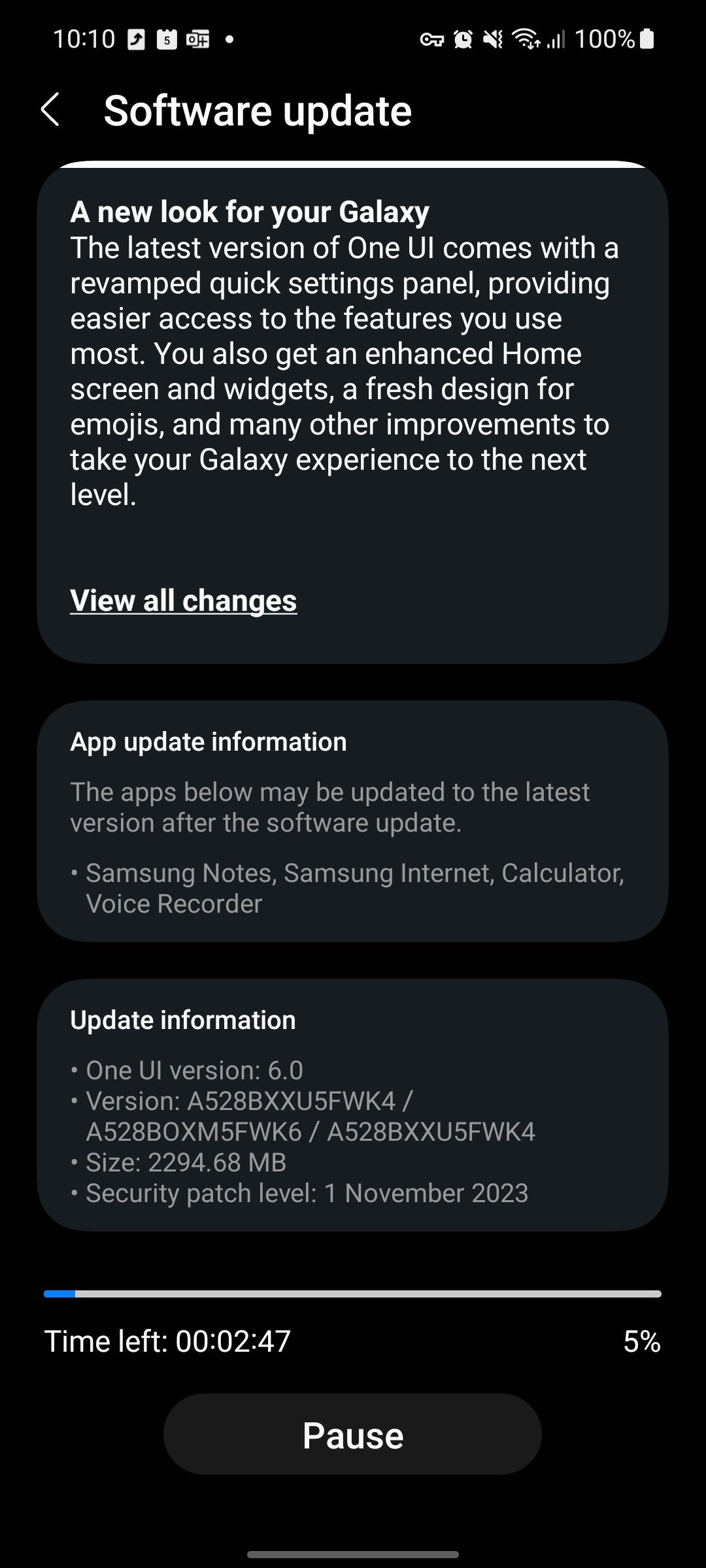The image features a predominantly black background concentrated at the top. At the very top left corner, there is a white number "5", possibly indicating the day. Adjacent to it are icons: a white key, a white clock suggesting an alarm, a white speaker icon indicating the device is on vibrate mode, and a battery icon at 100% charge.

Beneath this row of icons is a white arrow pointing to the left, next to the text "Software update" in white. Below this, a white line stretches across the screen. The main content is encapsulated in a black rectangle, which contains the following white text:

"A new look for your Galaxy. The latest version of One UI comes with a revamped quick settings panel, providing easier access to the features you use most. You also get enhanced home screen widgets, a fresh design for emojis, and many other improvements to take your Galaxy experience to the next level."

Underneath this, the text "View all changes" is underlined.

The next section, titled "App update information" in white, states that certain apps may have been updated post-software update, listing apps: Samsung Internet, Calibre, and Voice Recorder.

Following this is another section titled "Update information" in white, detailing:
- One UI version: 6.0
- Version: A52ABXXU5FWK4 / A52ABOXXM5FWK6 / A5228BXXU5FWK4
- Size: 2294.68 MB
- Security patch level: 1, November 2023

The bottom of the image displays additional information: "Time left 0.02.475%", followed by the word "poll" in white.